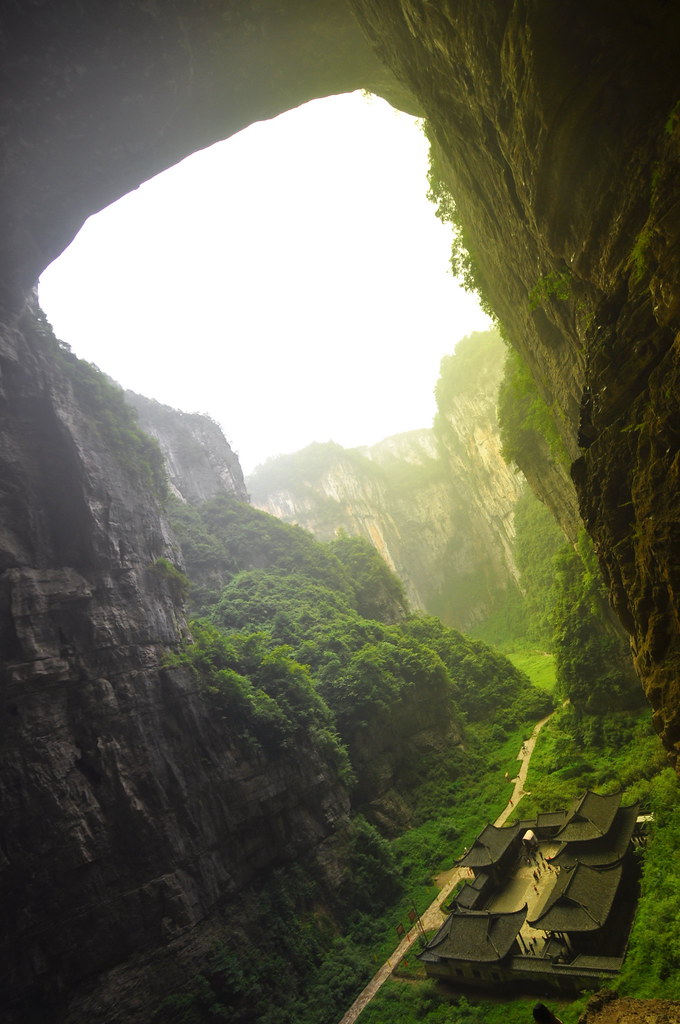This aerial photograph captures a breathtaking view of a temple complex nestled at the base of a lush, verdant canyon. The temple, comprised of several interconnected buildings, sits majestically on a raised platform, with numerous people seen strolling through its spacious courtyard. Enclosed by towering rock walls, the sanctuary is bathed in natural shade, giving it a fresh and moist ambiance. The temple is accessed via a solitary road that winds past the compound and continues into the distance. The scene is framed through a natural opening in the canyon walls, revealing rugged cliffs in the background. The sky above is gray and overcast, with a palpable mist hanging in the air, adding a mystical quality to the serene landscape.